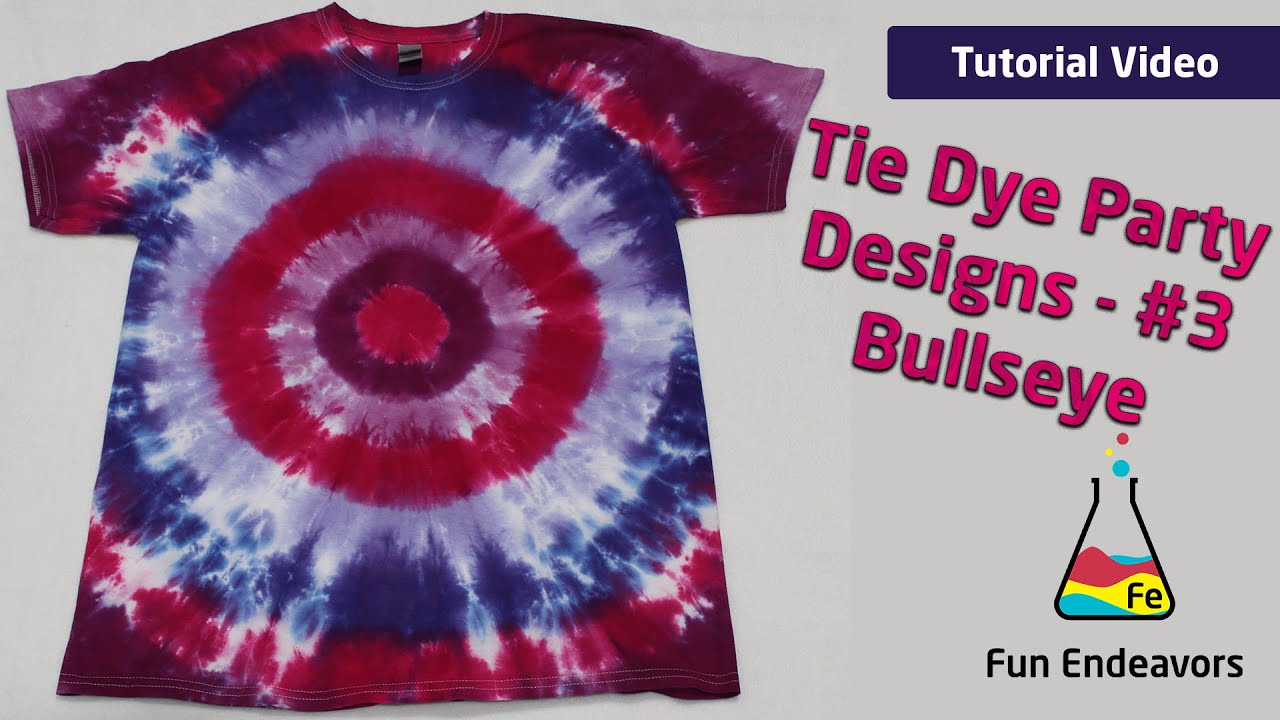The image is a horizontal, rectangular advertisement featuring a red, blue, and white tie-dyed t-shirt positioned on the left half, displaying a meticulous bullseye pattern. The background throughout is gray. On the upper right side, there is a dark blue tab with white text that reads "Tutorial Video." Below this, slanted pink text with a black outline says, "Tie-Dye Party Designs," followed by a dash and "Number Three: Bullseye." Beneath this text lies a logo consisting of a black-outlined beaker filled with red, yellow, and blue liquid, with bubbles of the same colors floating above. The initials "F.E." are inscribed within the beaker, indicating the company name, Fun Endeavors. This vibrant and colorful graphic appears to be promoting a tutorial video on creating the bullseye tie-dye design.